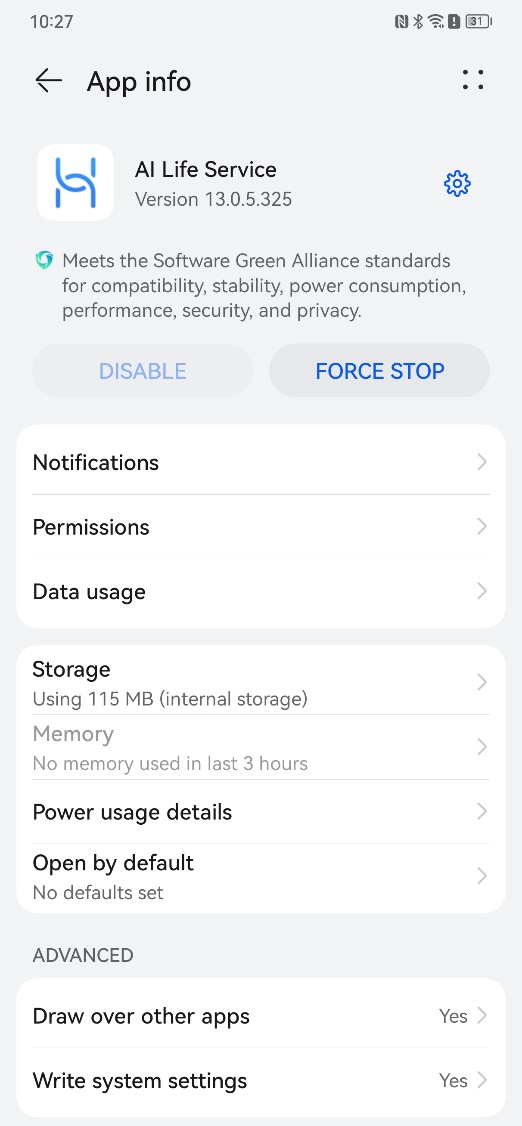This screenshot captures the 'App Info' tab for the 'AI Life Service' app, displayed against a grey background. At the top left, a backward arrow labeled 'App Info' directs users back to the previous screen. Centrally located just below is the app's icon, with the app's name 'AI Life Service' in black text situated to its right. The version number of the app is provided in grey just beneath the app name. Adjacent to the version number is a blue cogwheel icon, presumably for accessing additional settings. 

At the bottom of the information section, a certification states, "Meets the software Green Alliance standards for Compatibility, Stability, Power Consumption, Performance, Security, and Privacy." Below this certification, there are two action buttons: 'Disable' (which is greyed out and non-selectable) and 'Force Stop.'

Following this, there are three distinct white panels that categorize various settings:

1. **First Panel:**
   - **Notifications:** Options to configure how the app sends notifications.
   - **Permissions:** Controls to manage what permissions the app has been granted.
   - **Data Usage:** Insights into the app's data consumption.
   Each of these options is followed by right-pointing arrows for further expansion and adjustment.

2. **Second Panel:**
   - **Storage:** Information and settings regarding the app's storage usage.
   - **Power Usage Details:** Data related to the app's power consumption.
   - **Open by Default:** Indicates whether the app has a default action set, showing "No default set".
   Similar to the first panel, right-pointing arrows allow for further navigation.

3. **Third Panel: Advanced**
   - **Draw over other apps:** This setting is toggled 'Yes', allowing the app to overlay on top of other apps.
   - **Write system settings:** Also toggled 'Yes', permitting the app to modify system settings.

This meticulously detailed layout ensures users can efficiently manage and understand the various aspects and permissions of the 'AI Life Service' app.